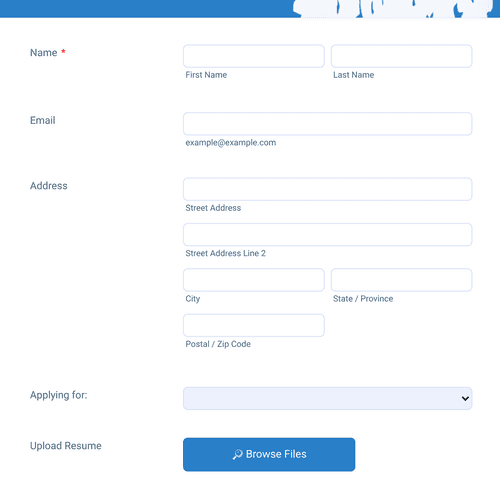The image depicts a vertically-oriented web page layout, approximately 30% taller than it is wide. At the top of the page, a blue banner gradually transitions into white towards the right, occupying approximately 5-10% of the total height. Below this banner, the background shifts to white, containing various form fields for user input.

Starting from the left, the first section is labeled "Name" accompanied by a red asterisk indicating a required field. This section consists of two horizontally-aligned input fields outlined in light gray. The first input field is labeled "First Name," and directly beneath it, the second input field is labeled "Last Name."

The second section is for the email address: it is labeled "Email" on the left with a single input field to the right. Below the input field, a placeholder example text reads "example@example.com."

The third section pertains to the address details. The label "Address" is followed by an input field for "Street Address." Beneath this, another input field is designated for "Street Address Line 2." Further down, an input field labeled "City" is provided, followed by another input field on the right labeled "State/Province." Below the "City" input, there is an additional blank area for further geographical information labeled "Country/Region."

The fourth section is for the job application, labeled "Applying for." It features a medium gray drop-down box with a downward-pointing black arrow, indicating that the user can select from various options.

The fifth and final section involves resume upload. It is labeled "Upload Resume," with a medium blue button to the right that contains white text reading "Browse Files." This button allows users to upload their resume directly through the form.